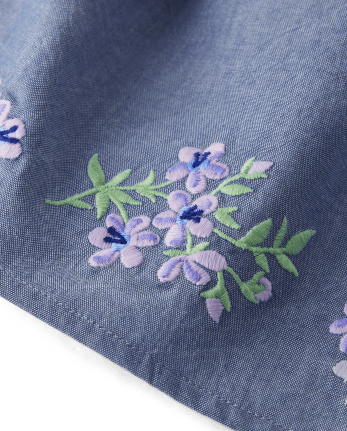The image displays a dark bluish-gray fabric reminiscent of denim but not quite like traditional blue jeans. The fabric is elegantly adorned with embroidered purple flowers that feature five to six petals each, with dark blue centers and delicate green stems and leaves. These floral patterns, which include flowers in various stages of bloom from buds to fully opened, are arranged prominently with some along the border and a detailed cluster of four flowers and three buds in the center. The lower left corner of the fabric is cut off at an angle, revealing a stark white background. The fabric appears slightly folded, casting subtle shadows that emphasize its texture and the intricate craftsmanship of the embroidery. The overall design is beautifully detailed and suggests it could be part of a finely crafted item such as a tablecloth or placemat.